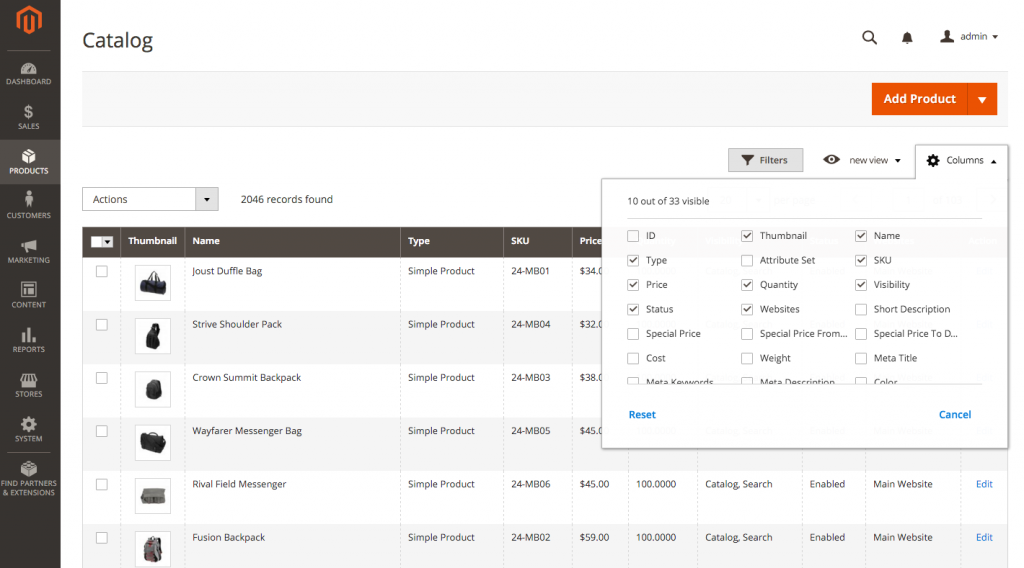The image captures a comprehensive page from a catalog interface, prominently displaying a record of 2,046 entries. At the top, the label "Catalog" is clearly visible, complemented by several functional options including an "Actions" drop-down, and buttons for "Filters," "New View," and "Columns."

A specific section indicates that 10 out of 33 fields are visible. These fields, many of which are checked, include: ID, Type, Price, Status, Thumbnail, Quantity, Websites, Name, SKU, and Visibility. Additional fields such as Special Price, Cost, Attribute Set, Special Price From, Weight, Meta Description, Short Description, Meta Title, and Color are available but not necessarily checked.

Towards the bottom, a list of products is featured, each accompanied by a brief description and images where applicable. The items listed include:
- A "Joust Duffel Bag," identified as a simple product.
- A "Strive Shoulder Pack," with an image of a black backpack-like item.
- A "Crown Summit Backpack," denoted as a larger black backpack.
- A "Wayfarer Messenger Bag" that sports a black handle.
- A "Rival Field Messenger," described as gray in color.
- A "Fusion Backpack," presenting a red and gray design.

The interface also boasts a blue "Reset" button and a blue "Cancel" button for user convenience. On the left side, the menu options are arrayed against a gray-colored background. The page itself is predominantly white and gray, accented by various product images enhancing the visual appeal while maintaining a clean and structured layout.